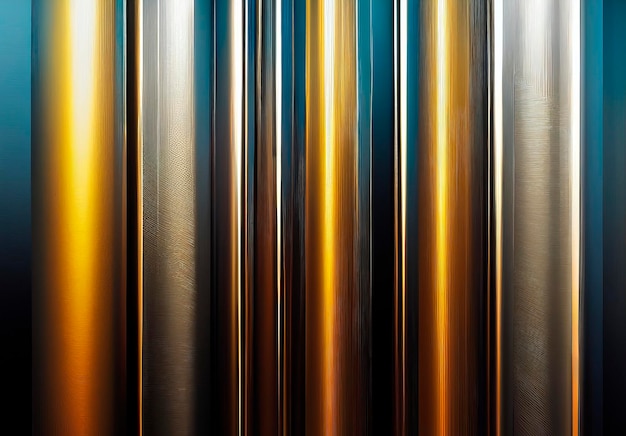The image features a vertical series of metallic stripes in varying depths and widths, which give the appearance of pipes on a teal background. The stripes have a glossy or metallic sheen, and the colors include turquoise, silver, gold, and copper. The pattern starts with turquoise, followed by silver, gold, and continues repeating these colors in different widths. Some stripes are wide while others are thinner, creating a varied visual texture. Light reflections accentuate the metallic quality of the stripes, making them appear like metal pipes rather than just painted lines. The sequence of colors and their reflective surfaces create a rhythmic pattern that spans the entire image, adding depth and complexity to the composition.